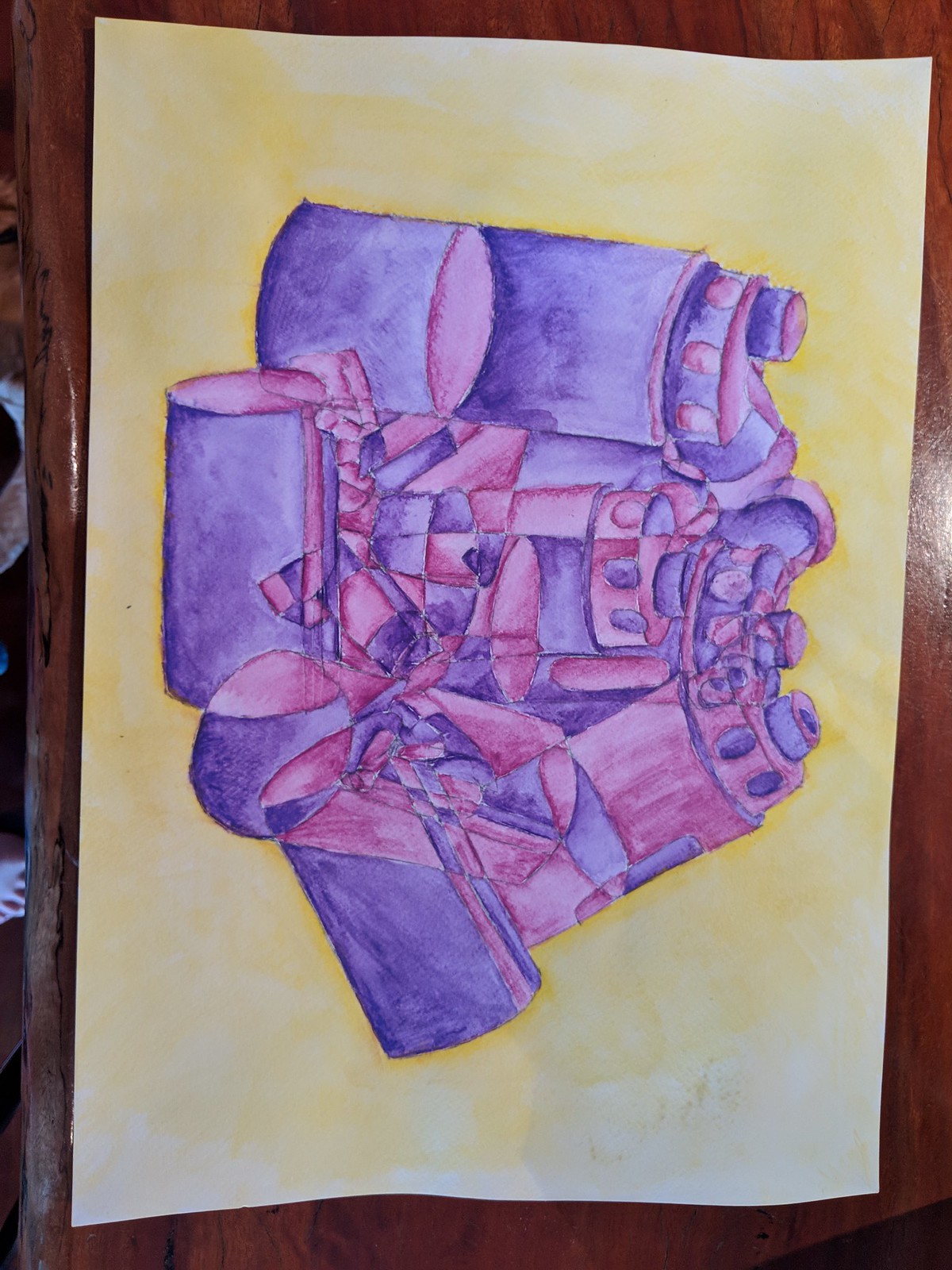The image is a graphic design illustration featuring a cluster of purplish-pink cylindrical shapes. These shapes resemble columns or pillars, leaning towards each other and interspersed with smaller cylindrical forms, creating a dynamic and intricate composition. The background is painted in a yellowish hue, which contrasts with the white paper on which the illustration is set. This paper appears to rest on a brown tabletop, adding a grounding element to the whimsical and abstract arrangement of the cylinders. The overall scene combines elements of modern graphic design with a vibrant and imaginative use of color and form.